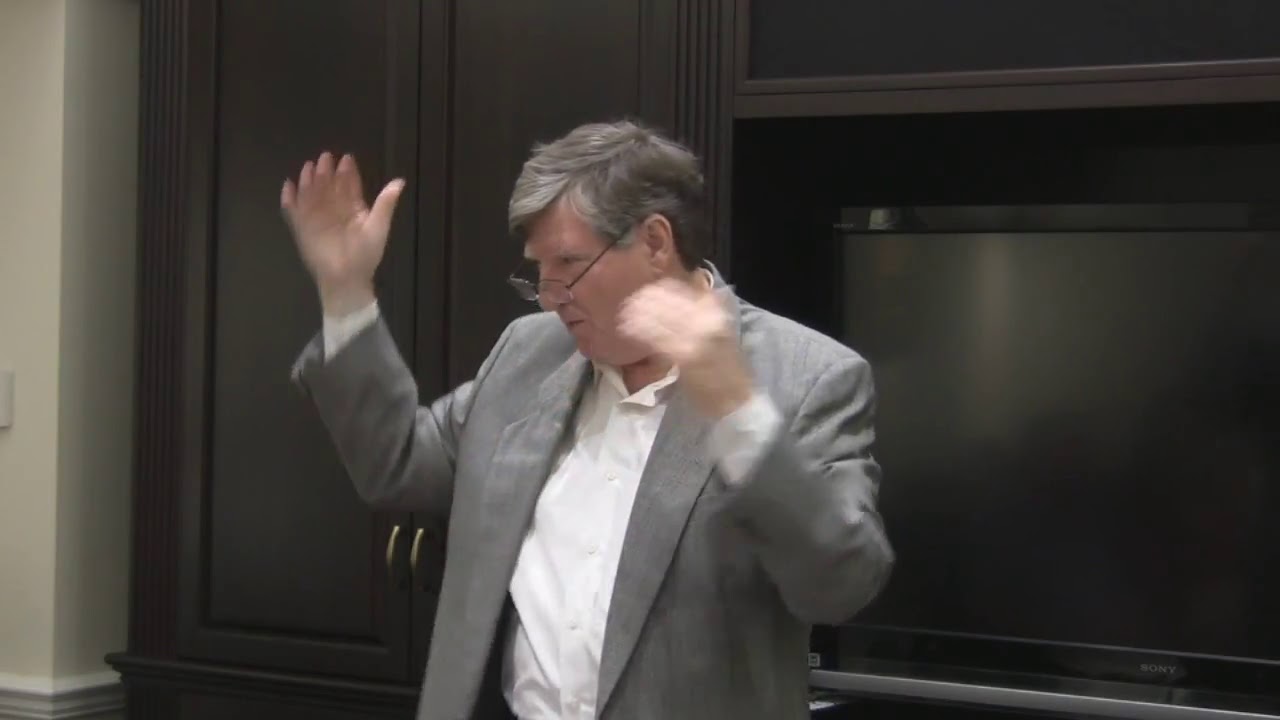The photograph captures an older man with light gray and white hair, prominently positioned in the center of an indoor office setting. He has fair skin and is wearing glasses, which are perched low on his nose. His attire includes a white open-collared shirt paired with a gray sports jacket. The man’s hands are raised and slightly blurred, suggesting he is engaging in animated conversation or teaching, while looking towards the right side of the frame.

The background features a wall unit consisting of a large dark brown or black wooden cabinet with closed doors on the left and a flat-screen TV, likely a Sony, on the right. The far left edge of the image shows part of a beige-white wall with a white lower section, adding contrast to the darker cabinetry that dominates the background.